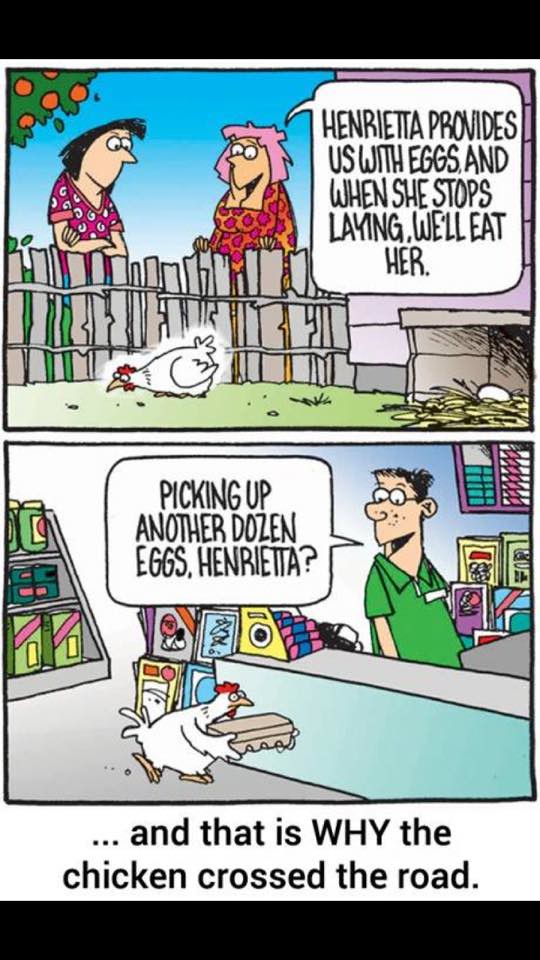This humorous vertical comic strip consists of two horizontal panels. In the first panel, two women are depicted standing behind a fence, looking at a chicken in a lush green yard. One woman, with pink hair, says, "Henrietta provides us with eggs and when she stops laying, we'll eat her." An orange tree is visible in the background, and an egg nest can be seen on the ground, enhancing the farmyard setting. The second panel below shifts to a grocery store scene where Henrietta, the chicken, is seen carrying a carton of eggs to the counter. A man with dark hair and glasses, presumably the cashier, remarks, "Picking up another dozen eggs, Henrietta?" The comic punchline at the bottom reads, "And that is why the chicken crossed the road."